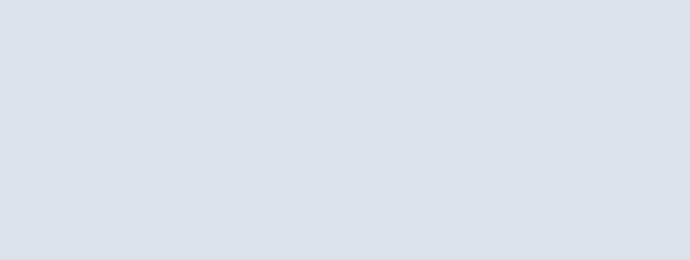The image is a completely blank, rectangular canvas, oriented in a landscape format. It extends longer horizontally from left to right than it is tall from top to bottom. The dimensions are moderate, neither very large nor very small in comparison to standard images. The color of the rectangle is a uniform light purplish-gray, with no variations or gradients in hue. There are no visible text, numbers, objects, or any other distinguishing features present within the image. The rectangle, which appears to be approximately an inch or two thick when viewed on the screen, is simple and devoid of any content or complexity, presenting a pure, uninterrupted expanse of light purplish-gray color.